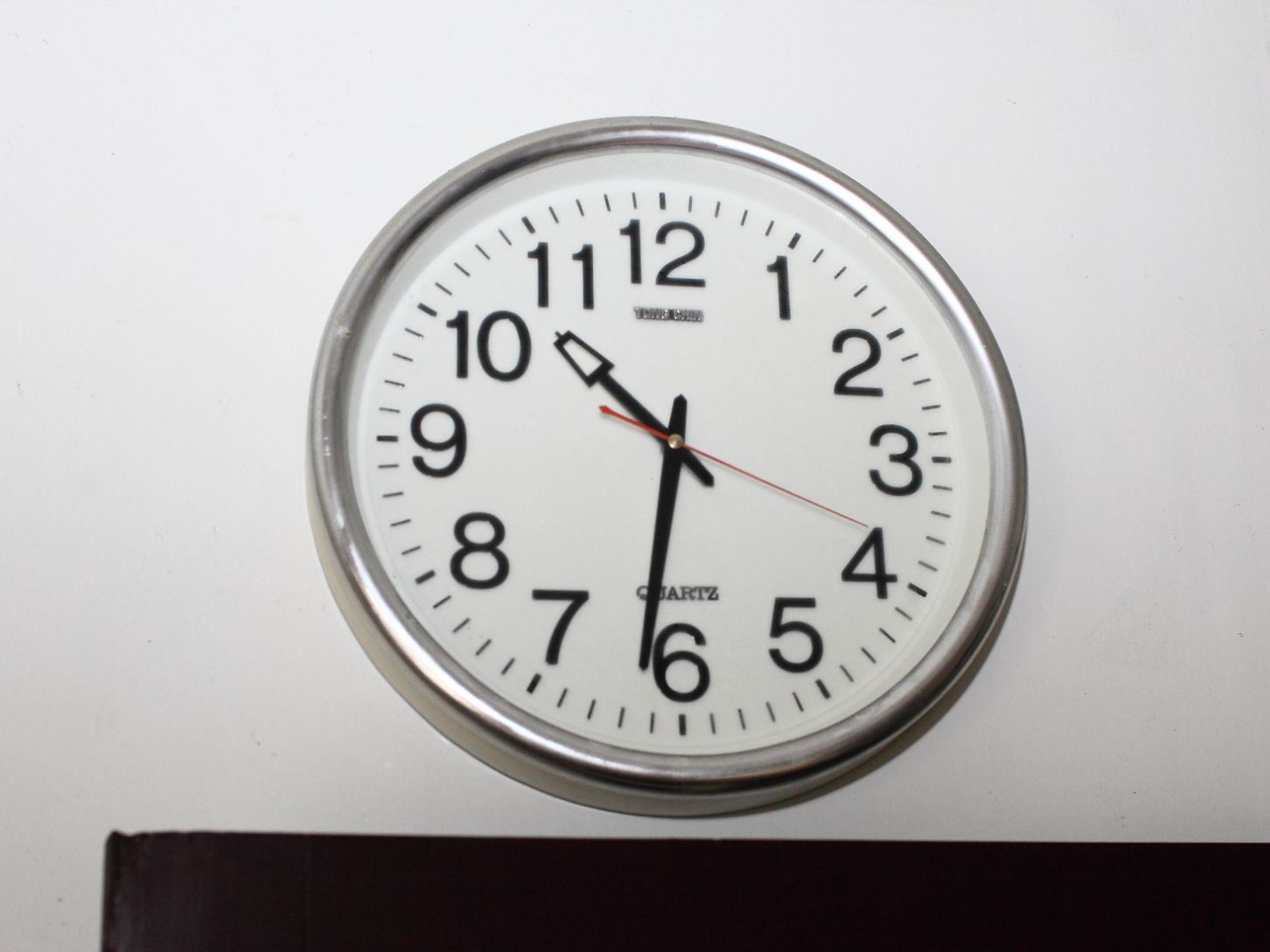A prominently displayed round wall clock, encased in sleek silver metal, adorns a whitish-gray wall. This sizable timepiece features a stark white face contrasted by bold black numerals marking each hour. Detailed minute markers encircle the face, contributing to its precision. The clock's three hands include the traditional hour and minute hands, complemented by a small red second hand. The hour hand is slightly broader with an open-style metal design, while the slimmer minute hand bears a pointed, slightly rounded tip. Though the clock bears a name, it is faintly visible, with "Quartz" clearly inscribed beneath it. The current time shows approximately 10:37 or 10:38. Below the clock, a dark object, possibly black or another dark shade, is discernable, though the monochromatic black and white nature of the photo makes it challenging to determine its exact color. The clock, with its meticulous design and clear functionality, stands out as a significant element in the room's decor.